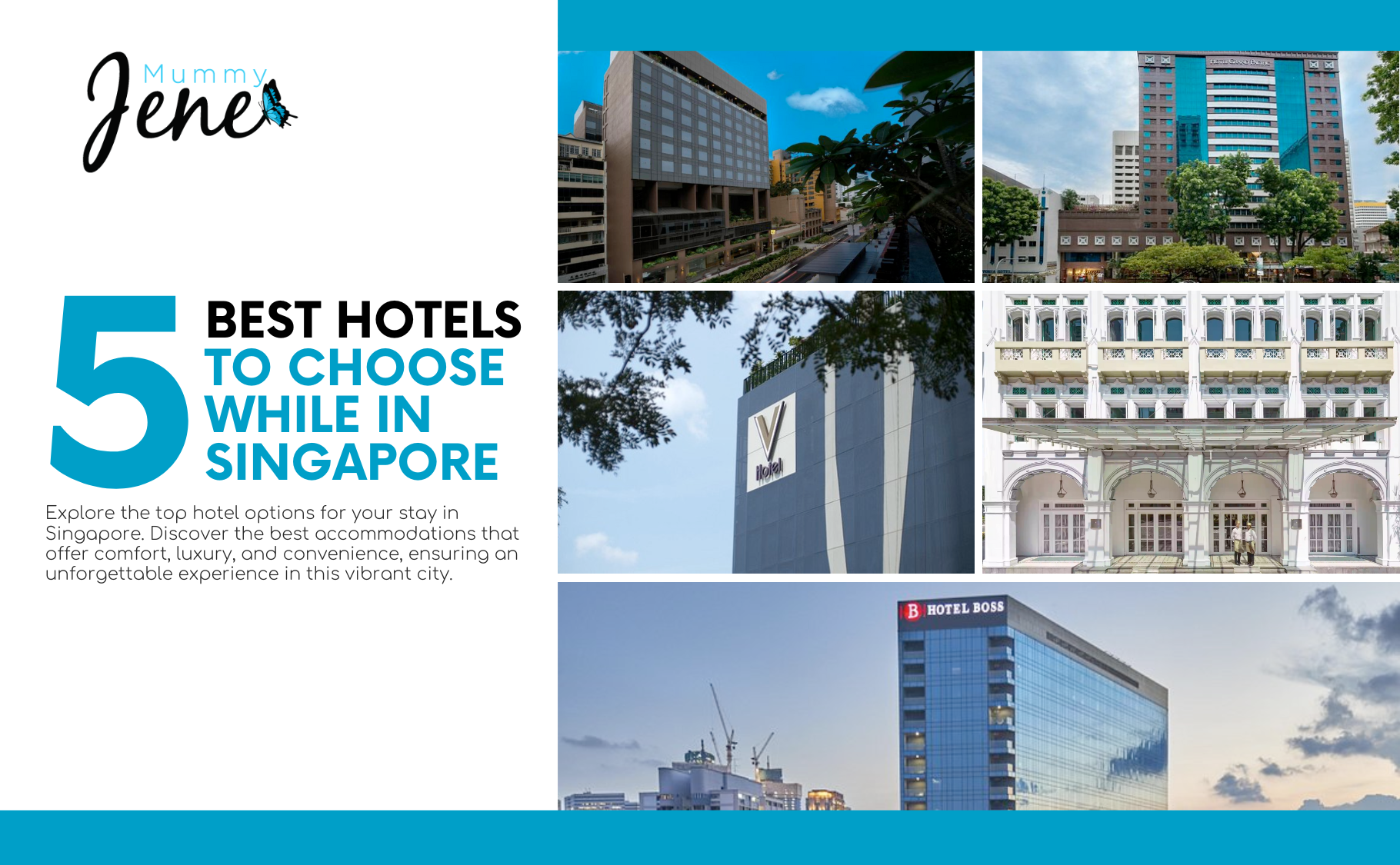This image is a snapshot of a webpage about hotels. In the top left-hand corner, against a white background, the text "Mummy Jean" is prominently displayed. "Mummy" is written in small, blue letters (M-U-M-M-Y), while "Jean" is in a more striking style, with a large, cursive capital 'J' followed by 'e', 'a', and 'n' in black. Adjacent to this, a teal butterfly with black-tipped wings adds a touch of elegance.

Below this logo, the headline reads "5 Best Hotels to Choose While in Singapore," with "5" and "to choose while in Singapore" in teal, and "best hotels" in black. Underneath, a smaller print elaborates: "Explore the top hotel options for your stay in Singapore. Discover the best accommodations that offer comfort, luxury, and convenience, ensuring an unforgettable experience in this vibrant city."

The page features five photos of hotels arranged in a column. The top two images are slightly smaller, showcasing various hotel exteriors. The middle two pictures also feature hotels, including a stylish building with a large capital "B." The bottom image is larger and highlights the "Hotel Boss" in full length. 

Overall, the composition and content suggest a well-curated selection designed to entice and inform visitors about premium lodging options in Singapore.